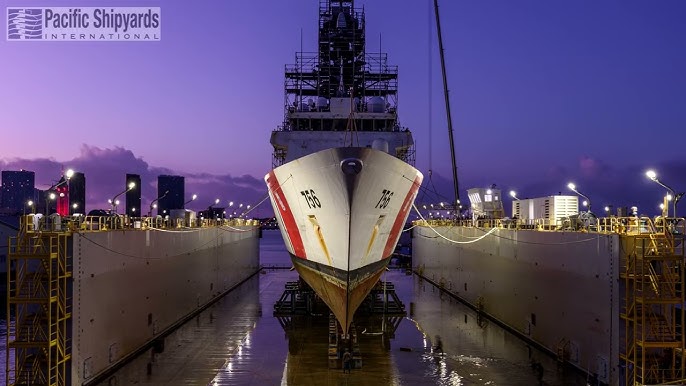A large ship, potentially a Coast Guard vessel, dominates the center of the photograph taken in the early evening, with the sky transitioning to dusk or dawn and skyscrapers visible in the distance. The ship, marked with the number 756 on both sides and adorned with vertical red stripes, is positioned within a docking station, suggesting it's either in a lock or completely out of the water for maintenance. The hull of the white ship is cradled between two tall cement or steel walls, each featuring yellow staircases. The foreground and surrounding area appear wet, hinting at recent activity or ongoing processes. Scaffolding is evident on top of the ship, underlining the maintenance work. The image is well-lit, capturing the scene brightly despite the dimming sky. In the upper left corner, the logo and name, Pacific Shipyards International, subtly assert the shipyard's identity, tying together the maritime setting with its industrial purpose.